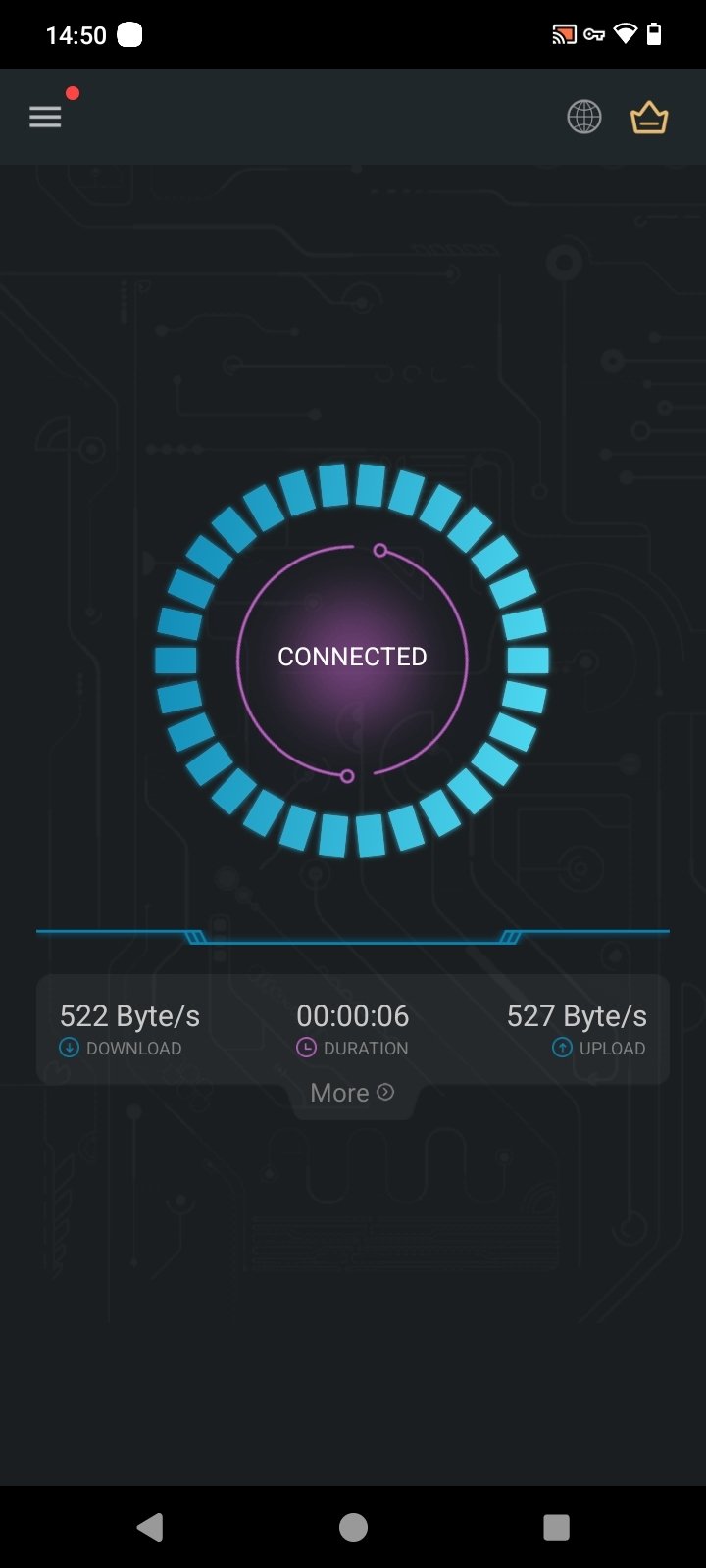Screenshot of a cell phone interface displaying a selection of VPN servers. The top of the screen features a black header bar with the word "Servers" written in white. To the left of "Servers" is a back arrow icon, and to the right, a refresh symbol. Below the header, there are two menu options, labeled "Free" and "Faster Servers."

Under these options is a white background section showing the available server list. At the very top of this section is an auto-selection feature labeled "Auto select the fastest one." Following this, a list of server locations is displayed vertically in the order: Germany, Singapore, Australia, India, Switzerland, Japan, South Korea, and the United Kingdom. Each server name is accompanied by the respective country flag and tagged as "VIP," indicating these are premium servers requiring payment. All server names are presented in English.